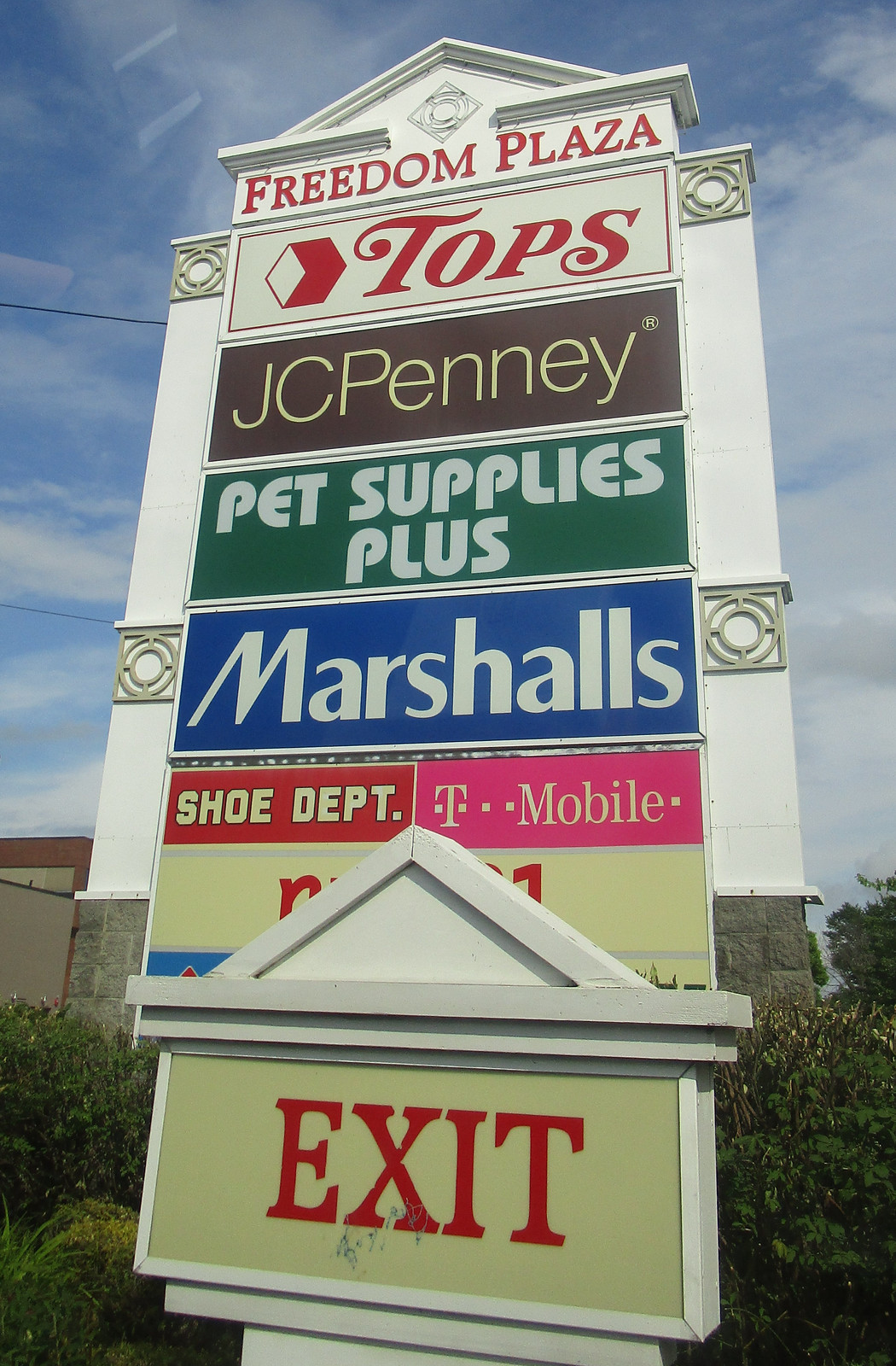The image features the welcome sign of Freedom Plaza, a bustling shopping center. Positioned prominently at the top, "Freedom Plaza" is displayed in bold red letters on a white background. Directly beneath, the well-known supermarket "Tops" is announced in striking red letters. Following this, the iconic "JC Penny" is written in white letters on a brown background, signaling its presence within the plaza. Further down, "Pet Supplies Plus" is distinguished by white letters on a green backdrop. Below this, the popular retailer "Marshalls" is presented in white letters set against a blue background. Adjacent to this, a red banner proudly indicates the "Shoe Department," and to its right, "T-Mobile" is highlighted on a pink background, showing the variety of services offered. Finally, a red "Exit" sign is situated at the bottom of the display. The sign is framed by a serene light blue sky adorned with subtle white clouds, and surrounded by lush green shrubbery.